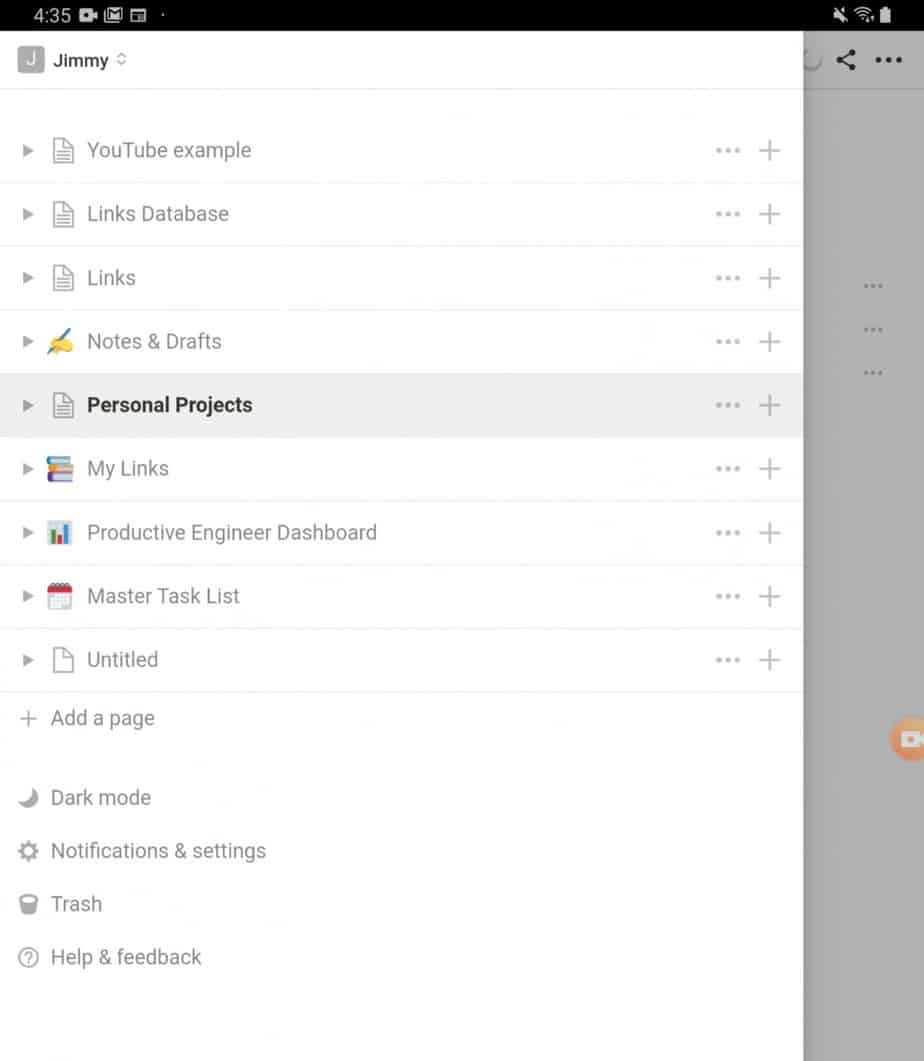The photograph depicts a screenshot captured from a mobile device in portrait orientation, featuring a clutter-free layout devoid of significant external borders. Dominating the top portion of the screen is a slender black status bar, which spans horizontally and contains several familiar icons: 

- A time display reading "4:35", 
- A camera icon,
- A Google Mail icon that indicates the presence of unread emails,
- A rectangular icon resembling a calendar or note pad, 
- A silent mode icon, 
- A Wi-Fi signal strength icon, 
- A battery icon that is fully charged, denoted by the solid white bar.

Below the status bar lies a large, vertically-oriented pop-up box occupying approximately 90% of the screen real estate. This box has a clean white background and is bordered at the top by a thin gray line.

In the upper left corner of the box, there is a gray square with a white letter "J" inside it, adjacent to the name "Jimmy" accompanied by up and down arrows. This section likely serves as a user identifier or profile selector.

Beneath this segment, a horizontal sequence of boxes laid out in rows appears, separated by fine gray lines. At the far right of this sequence, there are three vertical dots suggestive of additional options, along with an 'Add' button for further customization.

Aligned to the left within these horizontal boxes are various icons and clickable arrows, implying selectable options or menu items. The specific items listed include:
- YouTube examples,
- Links,
- Database,
- Notes and drafts,
- Personal projects,
- My links,
- Productive engineer,
- Dashboard,
- Master task list,
- Untitled,
- Add page.

Among these options, "Personal projects" is distinctly marked by a gray border, indicating it is currently selected or highlighted.